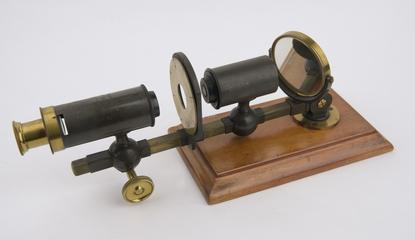This image depicts a vintage, antique device resembling a telescope, intricately crafted with a wooden base. On the left side, a dark gray and gold eyepiece extends from the main apparatus, which is designed for viewing. The eyepiece connects to a black body supported by several bars, leading to a small, gold-colored wheel near the front – possibly for adjustments. The device includes a small round mirror situated on the wooden platform to the right, encased in gold. This combination of materials and components gives the device an ornate yet functional appearance, highlighting its historical craftsmanship and scientific utility.